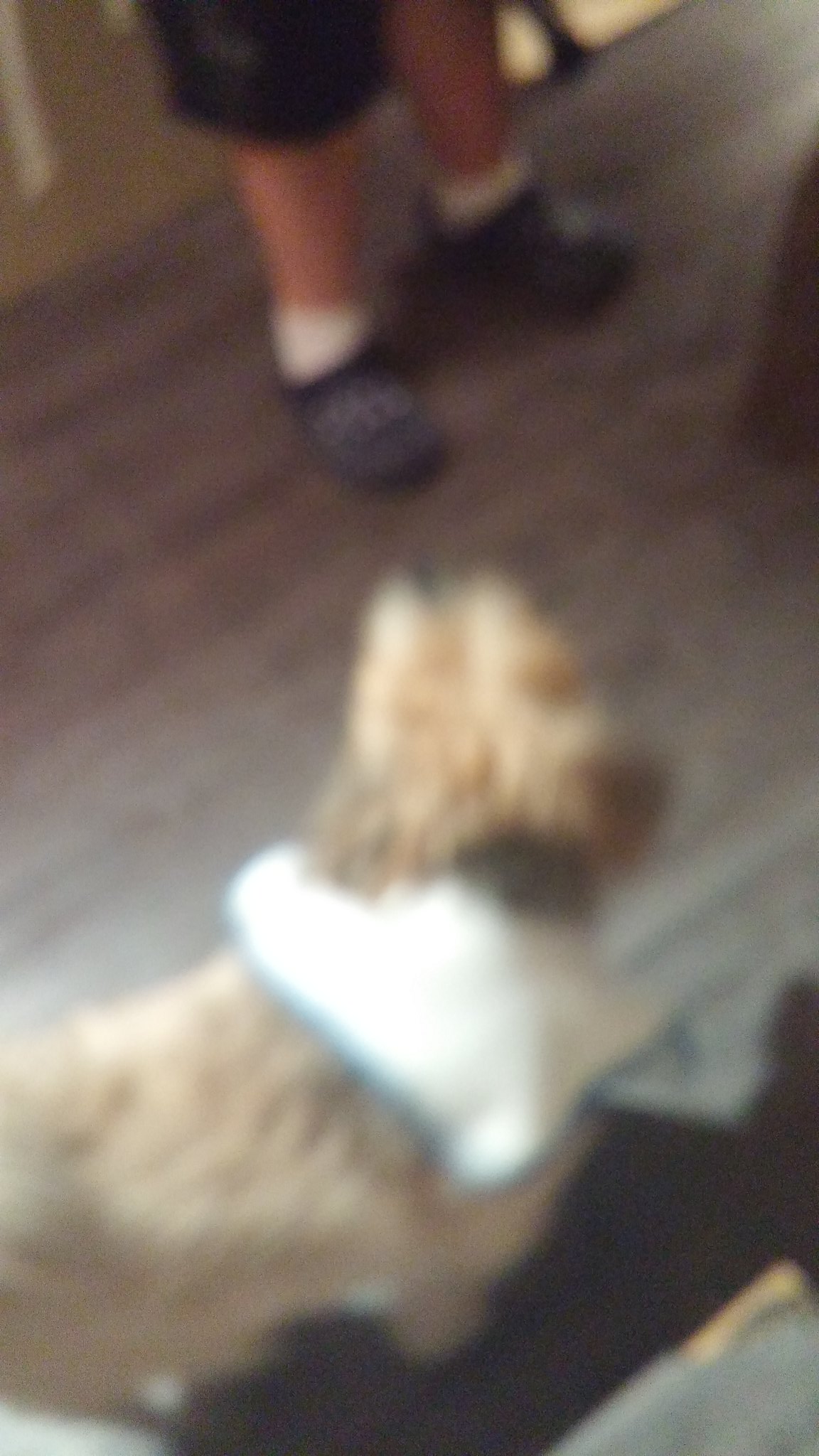The image captures a cozy scene on a slightly out-of-focus, grainy wooden floor. The focal point lies in a pair of visible ankles adorned with white socks and black slip-ons. Standing beside the feet is an adorable dog, featuring light fur and a white scarf with blue lines wrapped around its neck. The dog's head is particularly fuzzy, with its nose prominently sticking out, gazing intently at the person wearing the slip-ons. An evident shadow cast by the dog hints at a light source positioned at the top left corner, illuminating the lower left area of the scene.